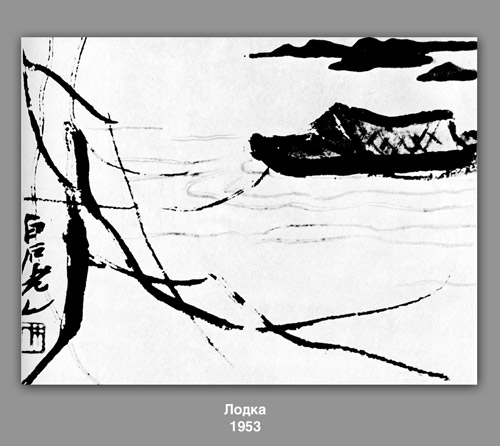This black and white painting, enclosed within a gray border with a thicker bottom edge, is a highly stylized depiction that combines bold and faint brushstrokes. Dominated by a predominantly white background, the artwork features various black lines and shapes, both dark and subtle, that evoke a sense of minimalistic elegance. The scene appears to show a body of water with light gray ripples, likely waves, contrasting starkly against the white expanse. At the center, a simplistic boat can be discerned, crafted in a manner reminiscent of traditional Chinese calligraphy, indicated by the sole use of black ink. Dark clouds occupy the upper right corner, balancing the composition. Additionally, the artwork includes multiple black rocks and stones, giving depth to the otherwise sparse landscape.

On the left side of the painting, faintly inscribed, are symbols resembling Japanese or Chinese characters, adding an exotic touch. Below this arrangement of ink, against the bottom gray border, is the text "n o a K a" in white letters, with the year "1953" indicated beneath it—possibly written in Russian script. The overall texture, the placement of elements, and the monochromatic palette converge to create a tranquil yet enigmatic representation, capturing the essence of an abstract marine scene.